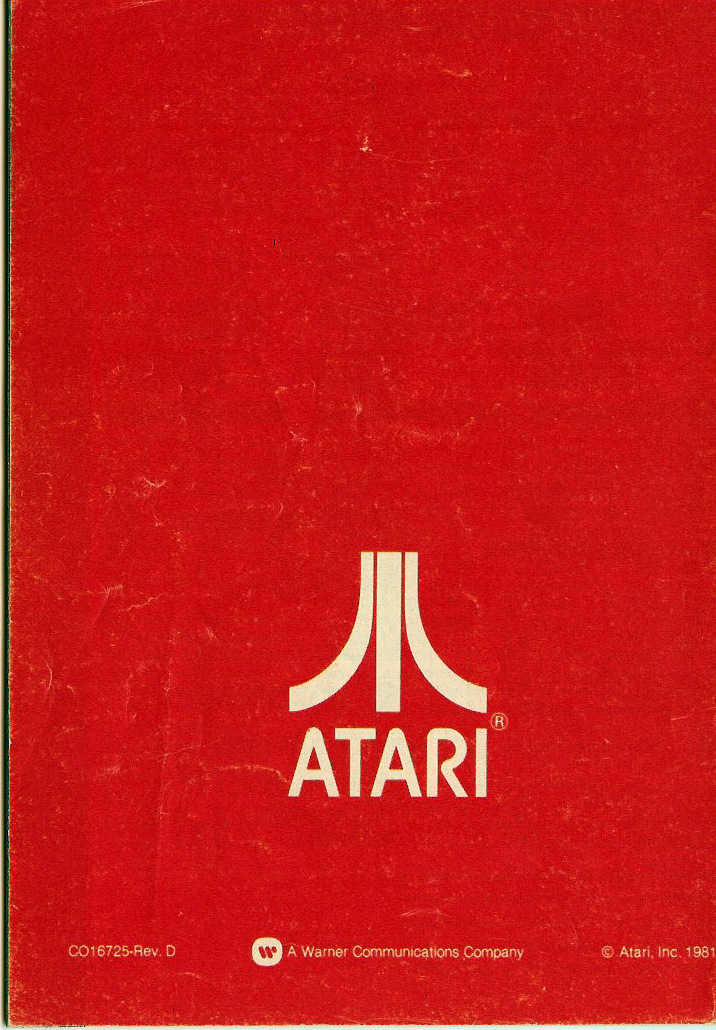This image showcases the back of a worn and faded red cardboard box, rectangular in shape and standing vertically. Prominently displayed in the center is the classic Atari logo, featuring a thick, straight white line flanked by two curved lines, giving it a stylized and distinctive look. Below the logo, in bold white letters, "ATARI®" is prominently printed, with the registered trademark symbol (®) positioned to the lower right of the "I". The red background appears solid but is scratched and discolored with signs of age and wear.

At the bottom of the box, in small white text, is the code "CO16725 REV.D" on the left-hand side. Further down, the text reads "Warner Communications Company" alongside the Warner Brothers logo, and "© Atari, Inc. 1981." The box, presumed to be from the early 1980s, seems to have been well-used, bearing visible wear and tear that hints at its age and the history of use.